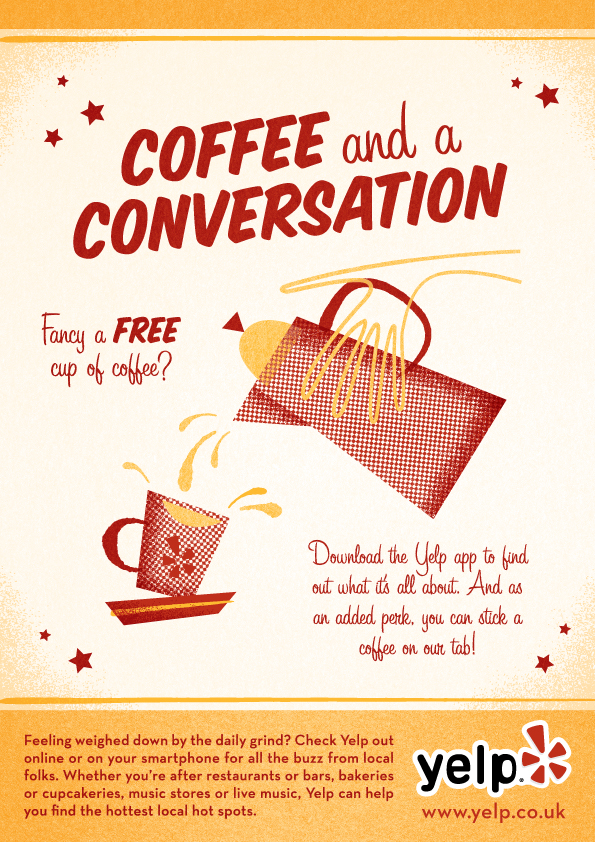This image is an illustrated, portrait-oriented promotional ad for Yelp, featuring a blend of typography and graphic design. The ad is primarily cream-colored with an orange gradient at the corners and consists of three main sections. 

At the very top, a horizontal orange strip holds bold white text reading, "coffee and a conversation," flanked by red stars. Below this, the central cream-colored section showcases a detailed illustration of a woman's hand outlined in gold, holding a red textured tea kettle with a gold dome lid and dark red handle. The kettle is pouring a gold liquid, which splashes as it fills a teacup angled to the right. To the left of this imagery, red text reads, "Fancy a free cup of coffee?"

The bottom section of the ad is a wide horizontal orange strip with the Yelp logo in black and red situated at the bottom right corner. Above this, red text instructs, "Download the Yelp app to find out what it's all about. And as an added perk, there's a coffee on our tab!" The overall design combines vibrant colors and playful illustrations to convey its message in an engaging way.